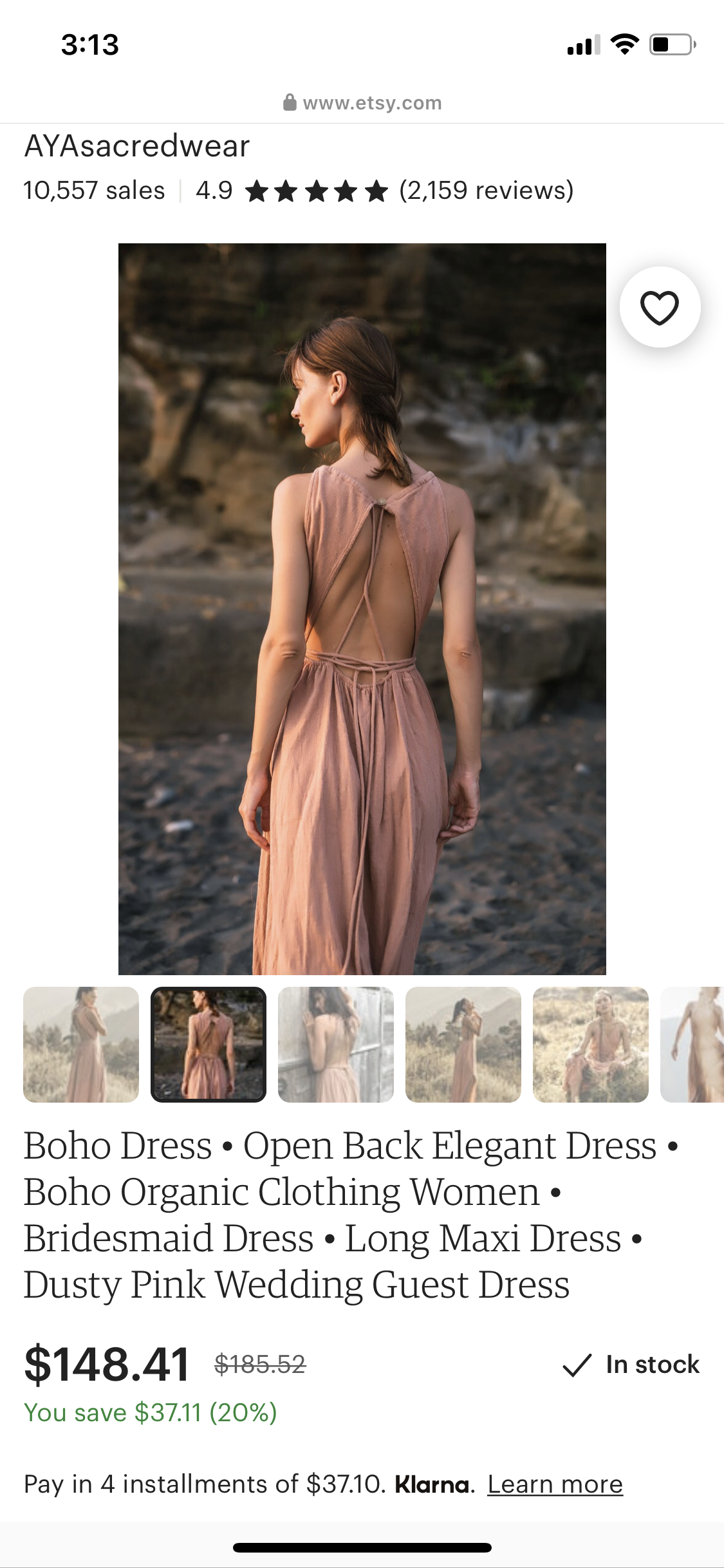The image is a screenshot from a cellphone, oriented vertically with a white background and black text. At the top of the screen, the status bar displays the time (3:13), Wi-Fi signal strength, and battery level. 

Centered below the status bar, in small text, is the URL: www.etsy.com. The main content shows a product listing for "AYA Sacred Wear" with a 4.9-star rating. 

The focal image features a woman wearing a long, open-back dress in a pinkish-brown hue. She is photographed from behind, standing on a beach-like terrain with sandy and earthy tones. 

Below the main image, there are several smaller thumbnail images showing different angles and positions of the same dress on the same woman. The second thumbnail from the left is highlighted, indicating it has been selected.

Beneath these images is a detailed description of the dress: "Boho dress, open back, elegant dress, Boho organic clothing women, bridesmaid dress, long maxi dress, dusty pink wedding guest dress." 

The price is listed at $148.41, and availability is confirmed with the text "In Stock" accompanied by a checkmark.